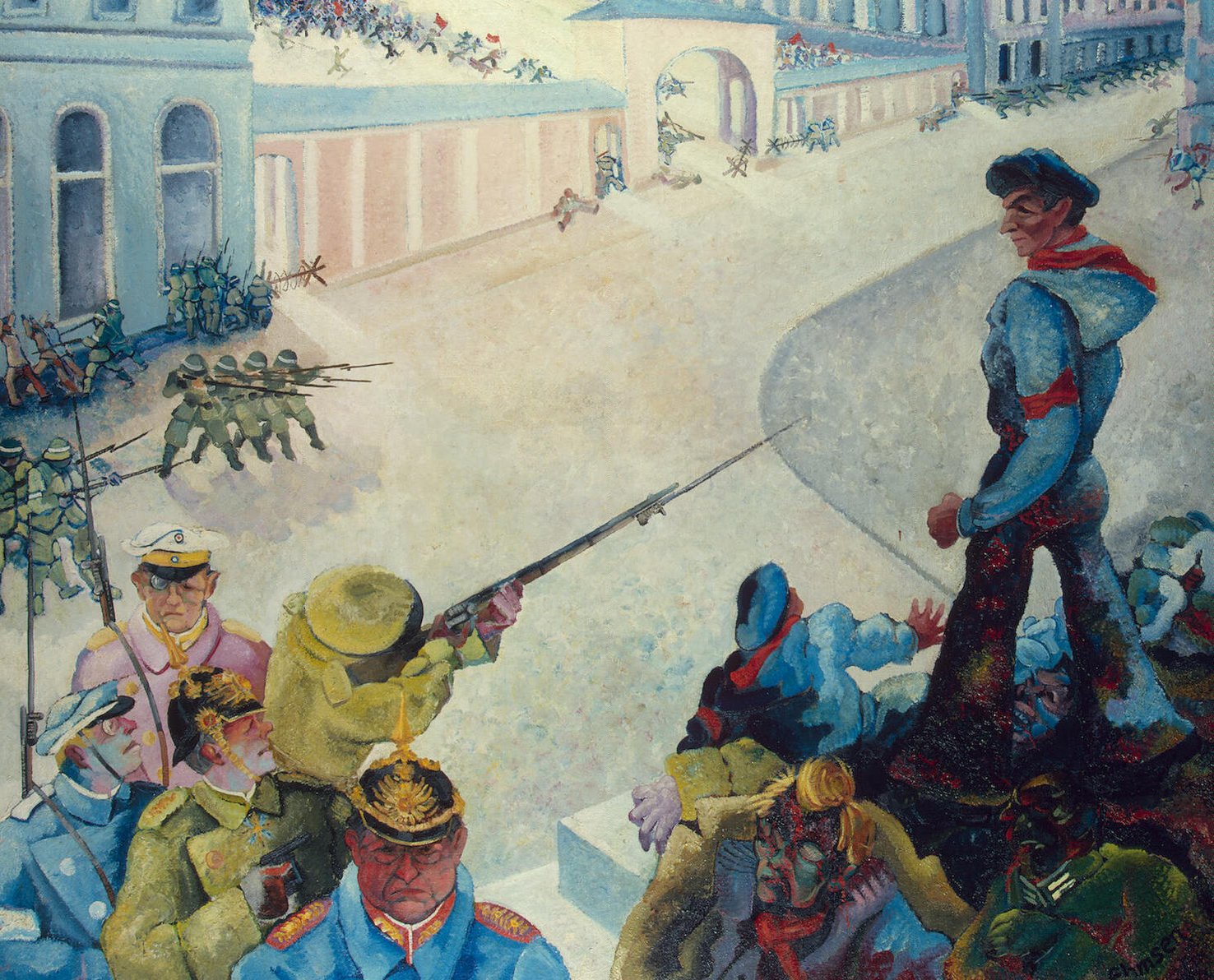This landscape-oriented painting, titled "Execution by Firing Squad of the Sailor Egelhofer" by Henrik Emsen from 1931, captures a dramatic scene of protest and resistance on a city street, likely set in 19th-century Madrid, Spain. Central to the image is a man standing on a platform on the right, wearing a blue jacket with a red ribbon tied around his arm, symbolizing his defiance. A soldier in a military uniform stands to the left, aiming a rifle with a bayonet directly at the man's head. Surrounding this soldier are others dressed in uniforms of various shades, some with helmets and others with hats, forming an ominous firing squad.

Further back, more soldiers can be seen lined up in formation, holding old-style rifles with bayonets attached. The backdrop features pastel-colored residential buildings with a large arched gateway at the center, adding depth and historical context to the scene.

On the bottom edge of the painting, a group of individuals in military garb mingles with civilians, some of whom appear to be trying to interfere with the imminent execution. This detailed and colorful art piece vividly portrays the tension and gravity of the historical event it represents, highlighting the stark contrast between the figures of authority and the lone figure of resistance.